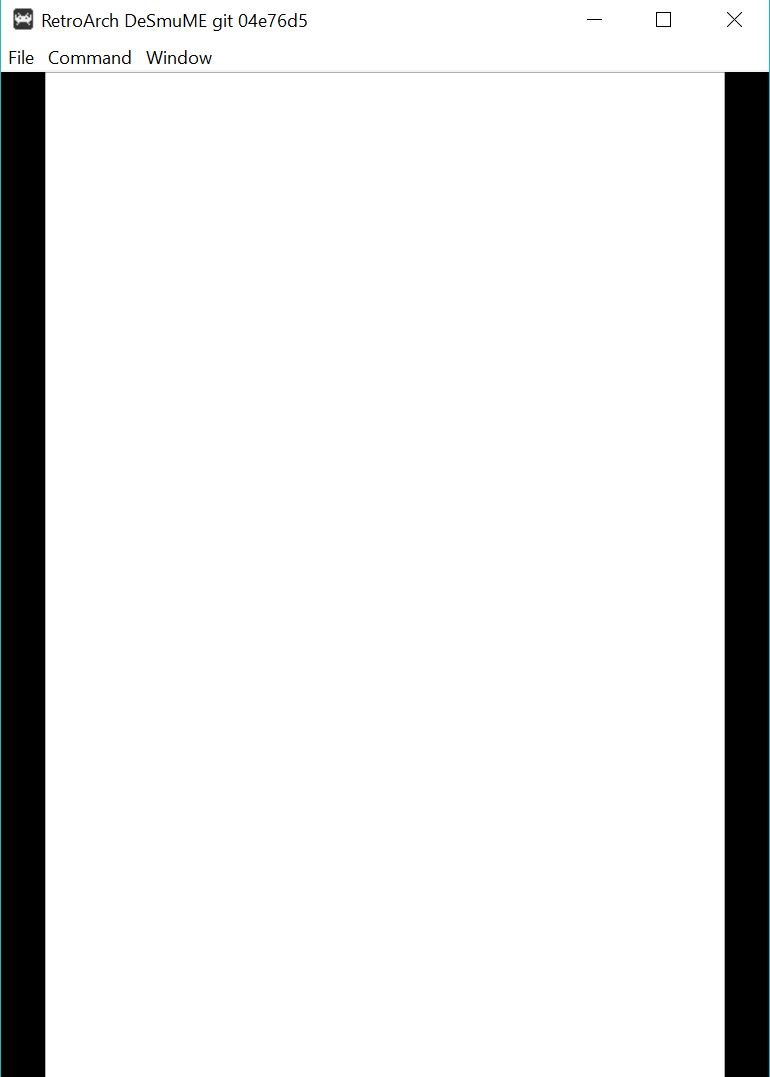**Screenshot of Settings Menu in RetroArch - Desmume Git**

The image captures the interface of a settings menu within the RetroArch emulator, specifically under the Desmume Git plugin. Dominated by a simple, clean design, the layout features an empty white canvas enclosed by black vertical bars on both sides. 

At the very top, a white rectangle with a black border spans the width of the screen. Inside this rectangle, positioned on the upper left, is an icon: a black square emblazoned with a classic white Space Invaders symbol. Adjacent to the icon, in sharp black font, is the RetroArch name stylized as "R-E-T-R-O-A-R-C-H," with a capitalized "A." Following this, the text continues with the specific plugin identifier: "D-E-S-M-U-M-E Git 04E76D5."

Beneath this header, three dropdown menus are aligned horizontally labeled "File," "Command," and "Window," all presented in black font, facilitating various functional commands.

In the upper right corner, typical window control buttons are displayed: a subtraction symbol for minimizing, a black square representing the maximize/restore function, and a black X for closing the window. The overall minimalist design underscores functionality while maintaining a nostalgic aesthetic.